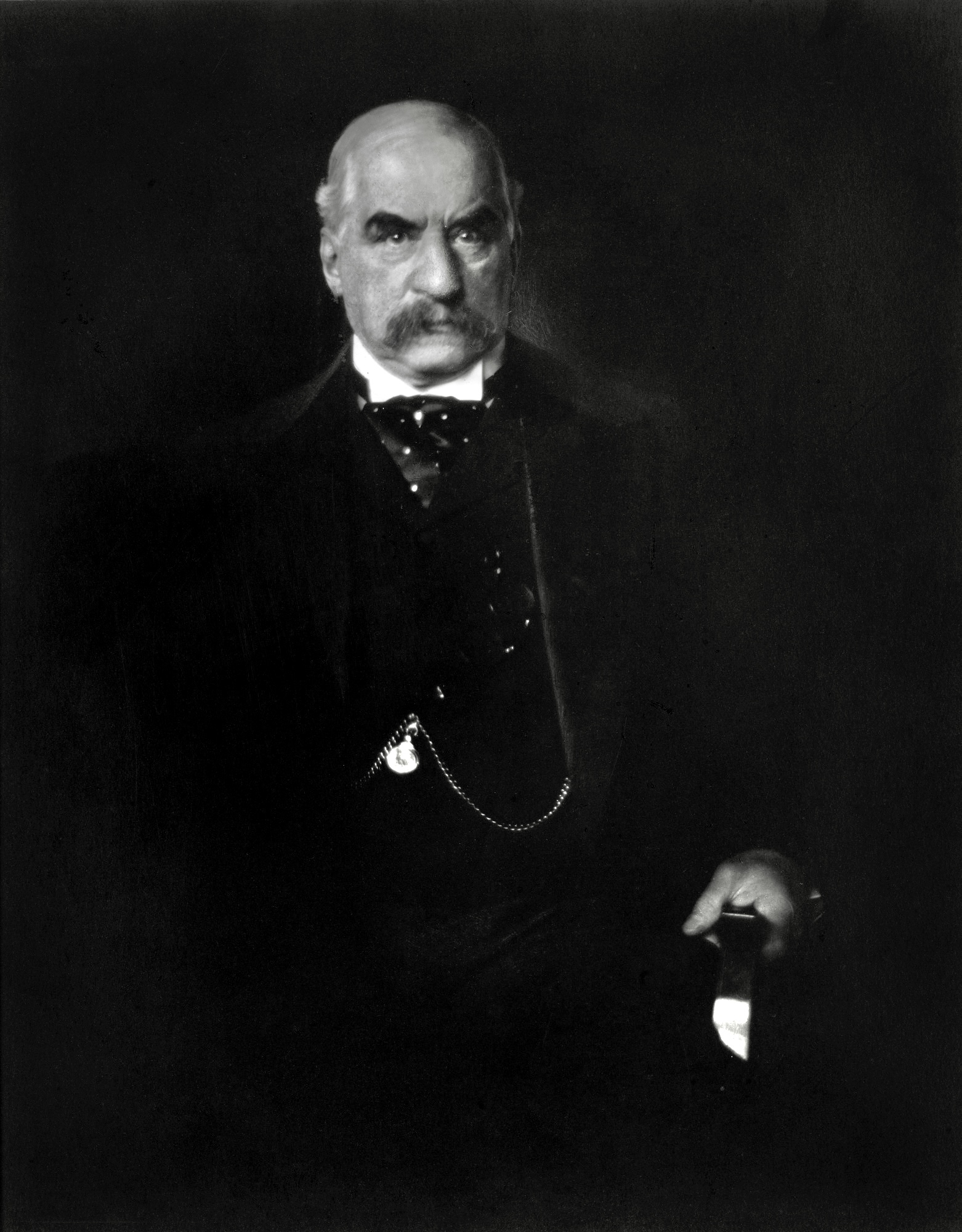A sepia-toned photograph from the 1800s features a stern-looking man with a distinguished appearance. He dons a black suit coat, adorned with a chain that stretches from the edge of the coat to a central button, suggesting it is likely from a pocket watch. Despite the image's age and lack of clarity, it's clear that he is wearing a white bowtie and a polka-dotted shirt underneath his coat. His thick mustache and white hair, styled in a neat comb-over, frame his face. The man's intense, squinting eyes exude an aura of anger or determination.

In his left hand, held sideways, is a dark gray kitchen knife or short sword, with its tip glinting white from a reflective light. On his left wrist, he appears to be wearing a wristwatch, and a pair of glasses seem to peek out from his left breast pocket. The overall dark ambiance of the photograph further enhances the man's commanding and mysterious presence.